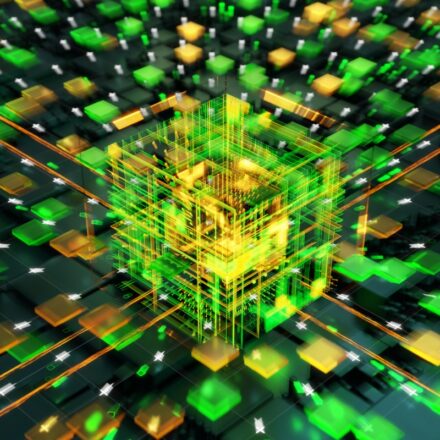This digital illustration showcases an advanced technological theme, centered around a semi-transparent, energy-formed cube. The cube's outer shell is primarily green, interwoven with yellow and orange lines, and encloses a smaller, brighter yellow cube. The intricate details resemble a high-tech processing unit or circuitry model. The background is a sleek black surface adorned with glimmering, shiny squares. Orange lines run beneath the cube, extending to the image's edges, creating a dynamic flow. Additionally, the surface is dotted with tiny green and white squares, as well as elongated white star-like shapes, contributing to the overall complexity and futuristic feel of the composition.